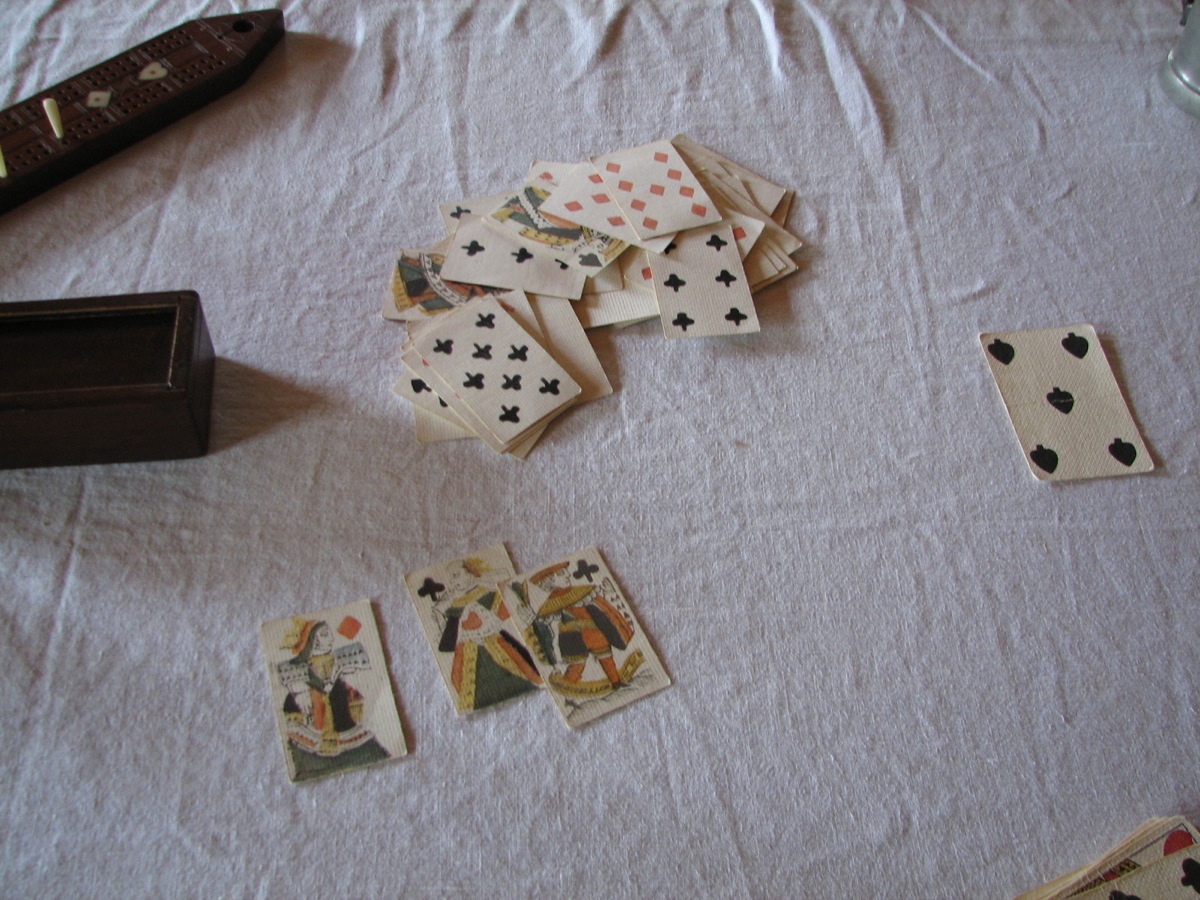The image depicts a collection of well-worn playing cards scattered across a very thin, wrinkled, white tablecloth. The cloth is exceedingly thin and white, with numerous prominent wrinkles at the top and more subtle creases throughout. In the top left-hand corner, there appears to be a game board, characterized by a brown rectangular base and a triangular top, perforated with several small holes, and a white peg inserted into one of them. Below this, a rectangular container, possibly metal or wood, is partially visible.

The playing cards show various suits with basic, rudimentary designs. Among the scattered cards, you can identify red diamonds, black clubs, and black spades. Notably, there is a solitary card on the right-hand side featuring five black spades oriented downwards.

In the foreground, several royal cards are prominently displayed. From left to right, there is a Queen of Diamonds, Queen of Clubs, and possibly a Jack of Clubs. The queens are illustrated wearing intricate, medieval-style gowns adorned with black, yellow, and red patterns, while the jack sports similarly colored attire. Additionally, parts of other cards are visible in the bottom right-hand corner, partially obscured by the arrangement.